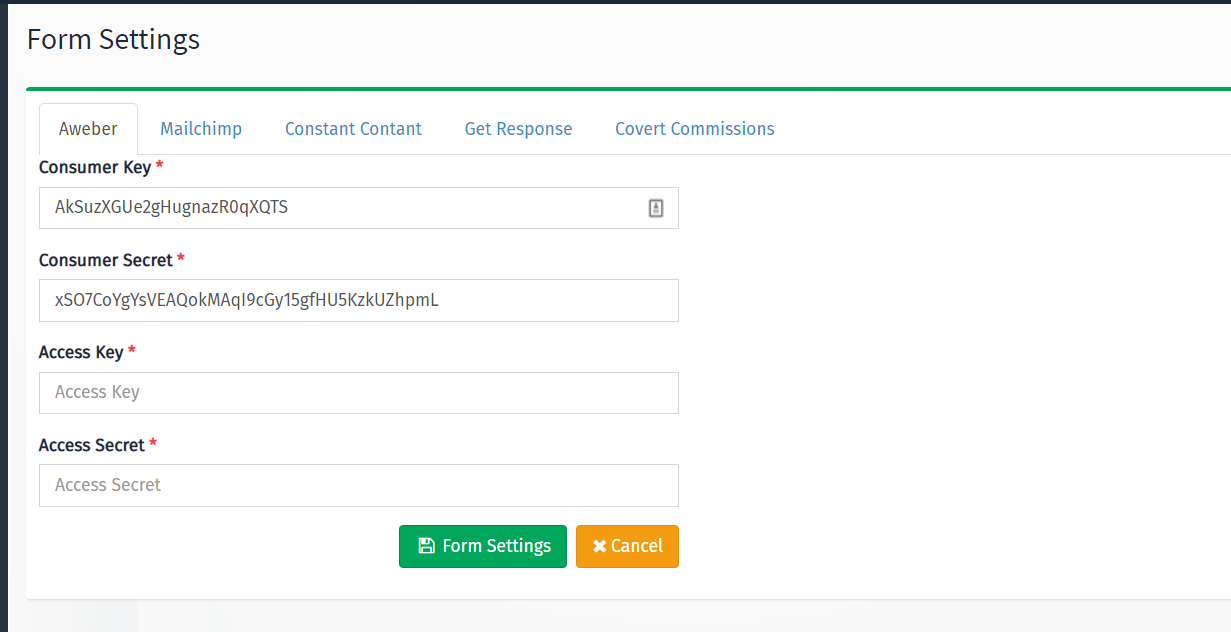This image depicts a web page featuring a form intended for MailChimp integration. The background of the page is white. At the top left corner, there is the heading "Form Settings". Directly underneath this heading is a thin, elongated green bar. Below this green bar are navigational tabs for different sections of the website.

The currently selected tab is "AWeber", spelled A-W-E-B-E-R. Within this section, there are several form fields, each labeled and marked with a red asterisk indicating that they are required. The first field is for the "Consumer Key", and it is followed by the "Consumer Secret" field. Both of these fields are populated with lengthy keys or passwords.

Below these, there are two additional fields: one for the "Access Key", and one for the "Access Secret", both of which are also marked with a red asterisk. Unlike the first two fields, the "Access Key" and "Access Secret" fields are empty.

At the bottom center of the form, there are two prominent buttons. The button on the left is green and labeled "Form Settings", while the button on the right is orange and labeled "Cancel".

Additionally, there are several other tabs available for selection on this page, labeled "MailChimp", "Constant Contact", "Get Response", and "Covert Commissions". Each tab presumably leads to similar integration forms for the respective services.